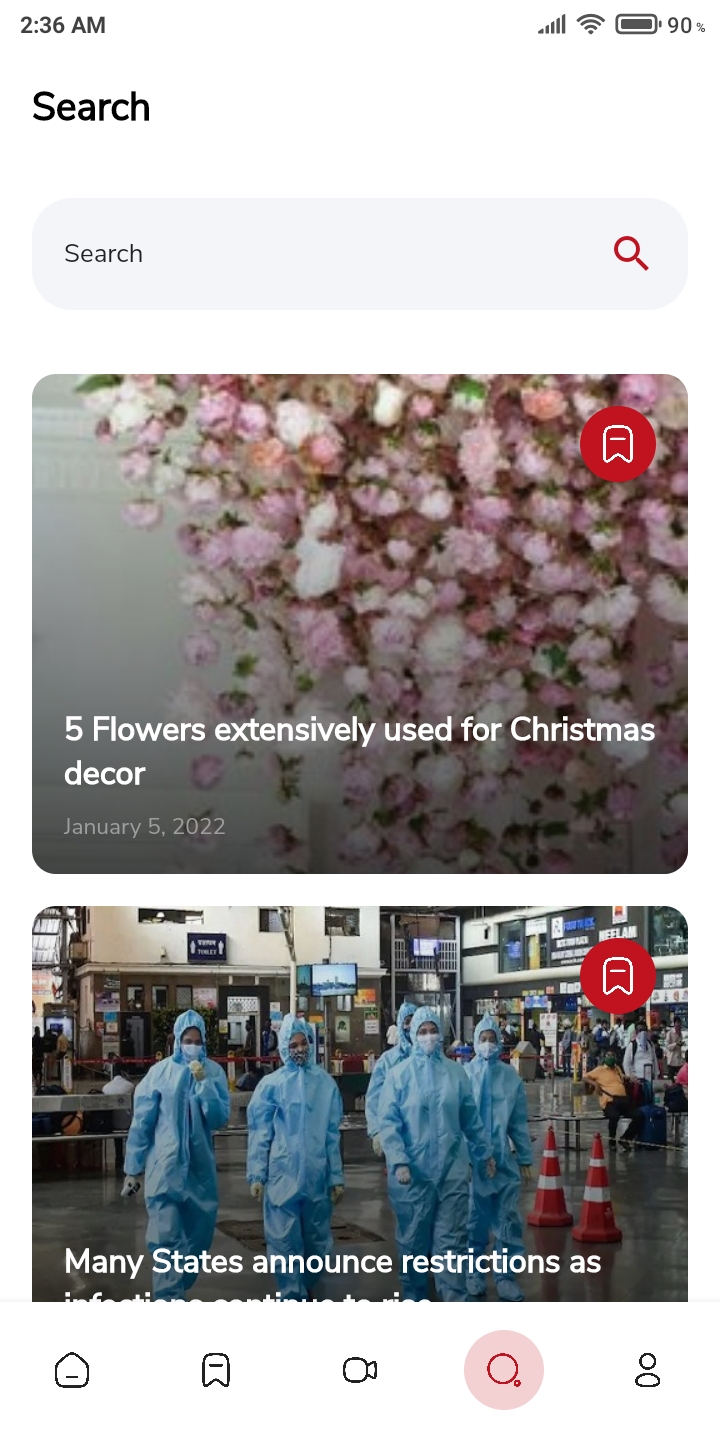The image shows a screenshot taken from someone's phone search results at 2:36 AM, indicated at the top left corner. Moving to the right, the status bar displays full signal bars, Wi-Fi connectivity, a 90% battery level, and a search icon. The search bar, located below the status bar, is gray with the word "search" and a red magnifying glass icon on the left.

The first search result headline reads, "Five Flowers Extensively Used for Christmas Decor," dated January 5th, 2022. In the upper right-hand corner of this article snippet, there's a red ribbon icon. The accompanying image features a bouquet of various flowers, including pink, white, and burgundy blossoms, accented with green foliage.

The second visible article snippet shows a group of individuals dressed in medical scrubs with masks and gloves, suggesting a healthcare setting. The partially visible headline states, "Many States Announce Restrictions As," with the remainder of the text cut off.